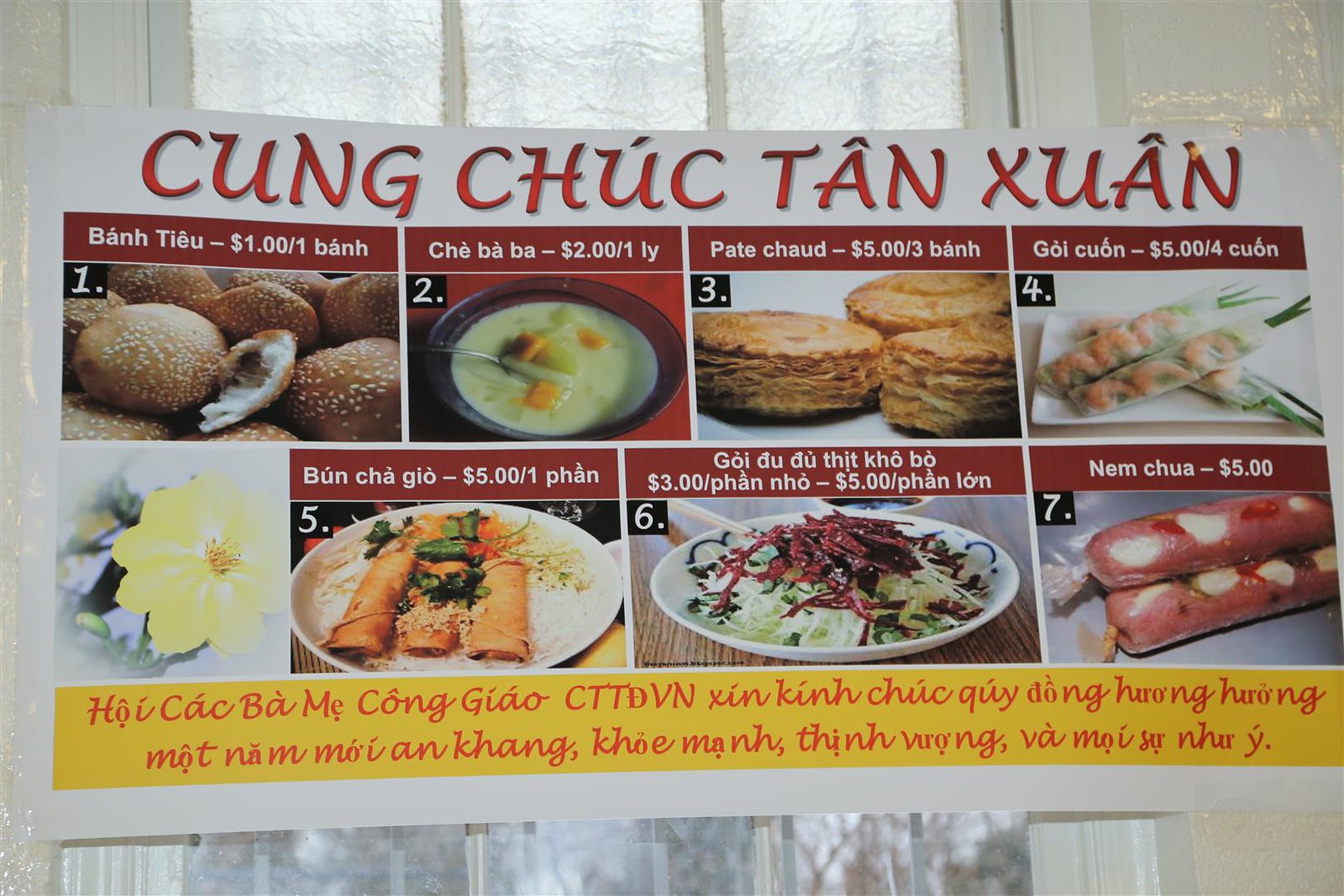The menu board of a Chinese restaurant is prominently displayed on a large piece of paper, taped to a white wall. Behind the menu board is a clear glass window with white window panes, allowing a glimpse of daylight or the scene beyond. At the top of the menu board, the name of the restaurant, "Kung Choo Tan Wan," is written boldly in both Chinese characters and English.

Below the restaurant's name, there is a neatly arranged set of eight tantalizing food images, organized in two rows of four. Each image is accompanied by a description written in Chinese, making the details accessible primarily to those who read the language. Despite the language barrier, you can distinguish several enticing dishes based on the provided transliterations and prices:

- Bun Cha Goi for $5
- Nim Chua for $5
- Ate Chua for $5
- Ban Tu for $1

The visual presentation suggests a variety of culinary delights, likely featuring an assortment of breads, soups, rolls, and salads, representative of traditional Chinese cuisine. The colorful images and descriptive layout on the menu board offer a tempting preview of the delicious options available at this authentic Chinese dining establishment.